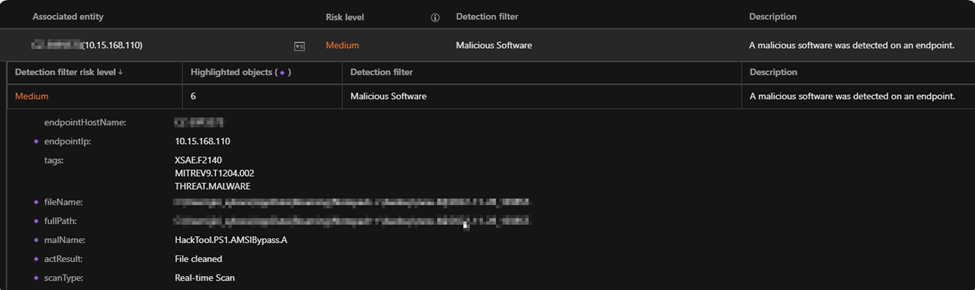The image depicts a detailed page written in extremely small font, resembling a tabular report. At the top of the page, the headers read "Associated Entity," "Risk Level," "Detection Filter," and "Description." The table appears to list information systematically.

Under the "Associated Entity" section, there is a blurred number followed by another numerical value. The "Risk Level" is marked as "Medium," and the "Description" notes that "Malicious software was detected on an endpoint."

Continuing with the table, the "Detection Filter" and "Risk Level" are highlighted once more, reiterating a "Medium" risk level. 

In the detailed breakdown:
- **Endpoint Names**: The names are blurred out.
- **Endpoint IP**: Displays the IP address "10.15.168.110".
- **Tags**: Includes identifiers like "xsae.f2140" and "mitrev9.t1204.002".

Further details:
- **Full Path**: Blurred.
- **File Name**: Recognizable text reads "hack.tool.ps1.amsibypass.a".
- **Scan Results**: File status is indicated as "cleaned".

Finally, the scan details specify the scan type as "real-time scan" conducted in real-time.